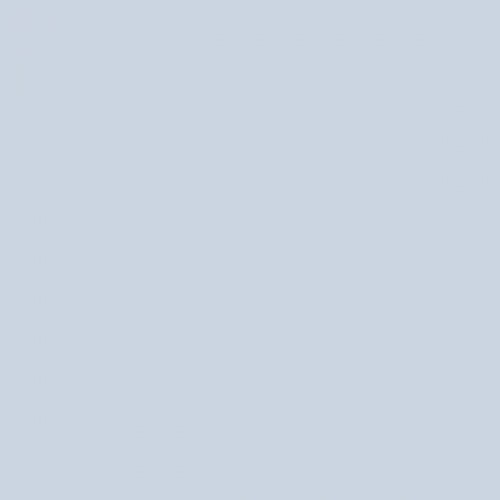A minimalistic image featuring a perfect square with right-angled corners and equal-length sides, filled with a subtle, nearly imperceptible blue hue. The solid color, a very light shade reminiscent of gray with the faintest hint of blue, spreads uniformly across the entire square. There are no gradients, transitions to other shades, or any variations in color intensity. The simplicity is further emphasized by the absence of any additional elements such as text, icons, lines, or designs. The image is purely a delicate, almost gray-tinted blue square, devoid of any content or overlays, offering a clean and unembellished visual.